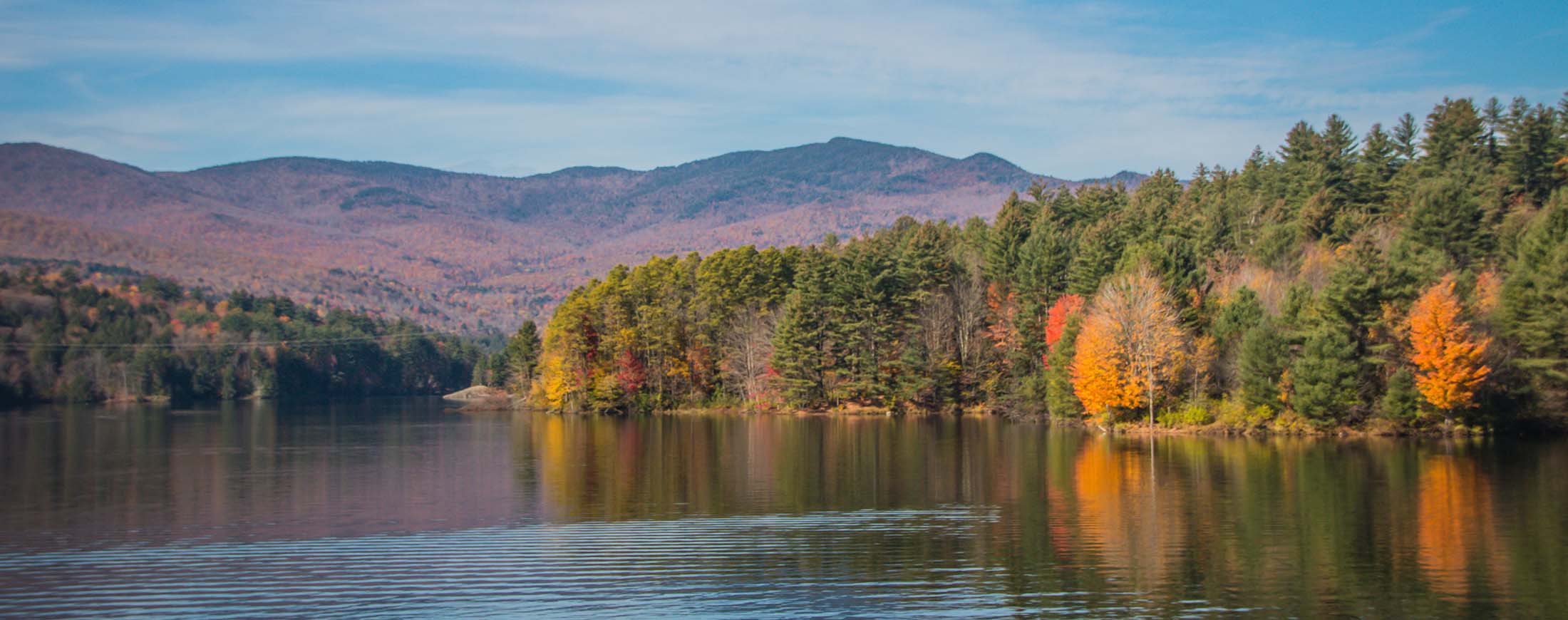The image is a wide panoramic view, approximately four times wider than it is tall, featuring a serene lake. The foreground showcases a calm, greenish lake reflecting the vibrant autumn leaves. Along the lakeshore, an abundant variety of trees are present, including pines, oaks, maples, and evergreens, with many beginning their transition into fall. The leaves are turning bright oranges, reds, and yellows, while some trees remain green and others appear bare. At the right, the tree coverage becomes less discernible. In the distance, a majestic mountain range rises, partially covered with trees transitioning to autumn hues. The top quarter of the image reveals a blue sky, scattered with faint, white clouds.